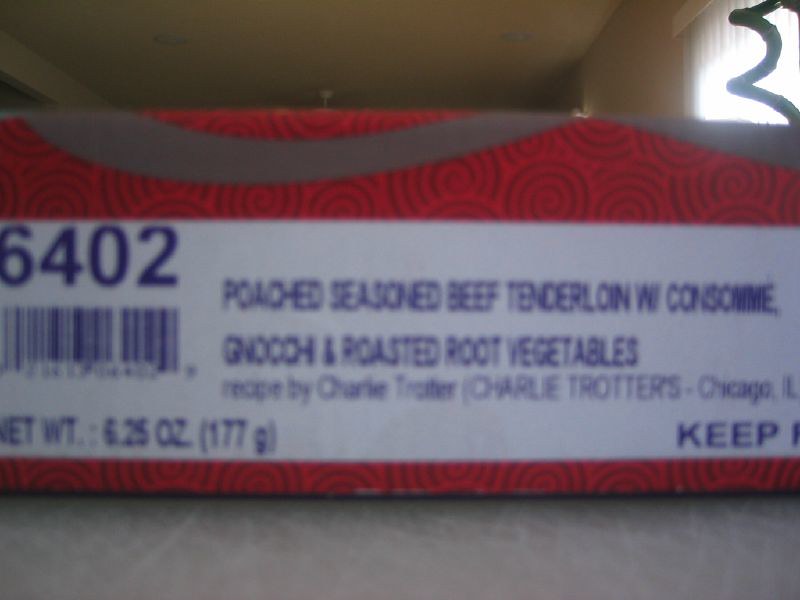The image depicts the exterior of a food packaging box, laying on its side. The box features a prominent red border running along the top and bottom edges, framing a central white label. In the top left corner of the label, the number "6402" is clearly visible. Directly beneath this, there is a slightly blurry barcode. The next line provides the net weight of the contents, which is "6.25 ounces (177 grams)." Centrally located on the label is a detailed description of the meal inside: "Poached, seasoned beef tenderloin with consommé, gnocchi, and roasted root vegetables." In the bottom right corner of the label, partial text is visible, starting with the word "Keep" followed by unclear content. Additionally, the label credits the recipe to "Charlie Trotter," specifying its origin as "Charlie Trotter's, Chicago, Illinois."